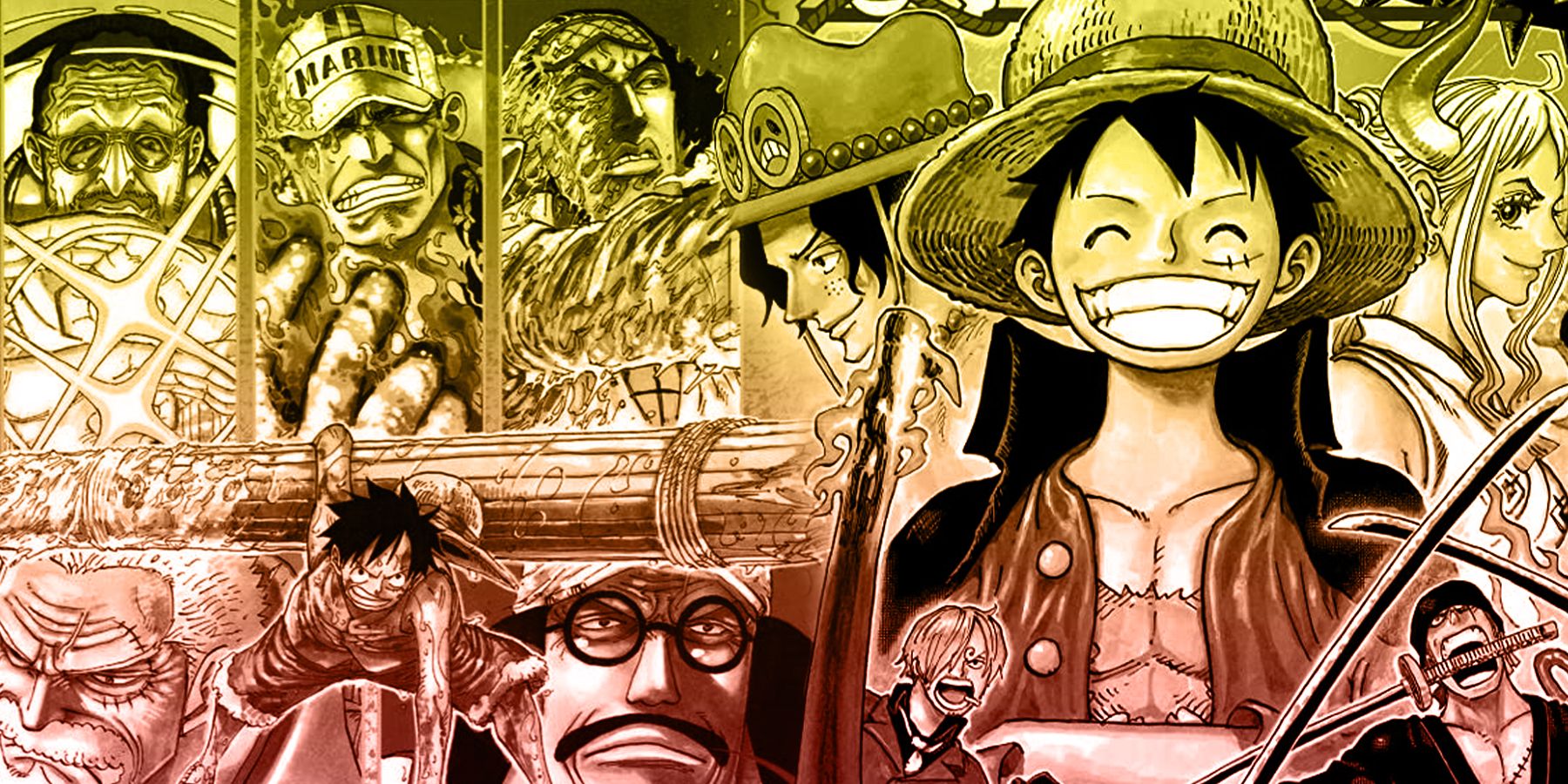This image is a detailed illustration from the anime show **One Piece**, featuring a diverse array of characters in a two-row layout with distinct colored borders: yellow on the top and red on the bottom, separated by a log. Central to the composition is the character **Monkey D. Luffy**, who is depicted wearing a straw hat, a red shirt, shorts, and holding a log on his back with one arm. To Luffy's left is an old man with white hair and a grim expression, while to his right stands a man with a thin mustache, black circular glasses, black hair, and a cap.

In the top left of the image is a man with black hair, partially obscured by light, making it difficult to see his wrinkles clearly. To the right of him stands another man, also donning a hat and somewhat covering his face with his hand. Adjacent to him is a bald man looking to the right.

On the right side of the image, Luffy appears again, this time with his straw hat firmly on his head, black hair peeking underneath, a big smile showing all his teeth, and his eyes closed. To the left of smiling Luffy is a man with black hair and a thin face, shown in side profile, looking to the left. To Luffy's right is a light-haired woman, also in side profile, with a smirk on her face.

Below these characters, towards the bottom left, is a blond-haired man with his mouth open, and next to him is another man, also with an open mouth, holding a sword handle between his teeth. The overall vibrancy and variety of expressions capture the dynamic and adventurous spirit of **One Piece**, showcasing a mix of intense action and joyful camaraderie.